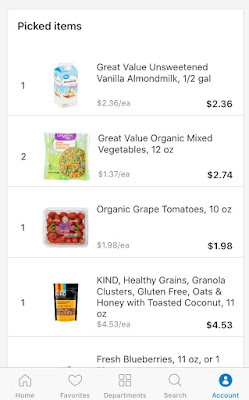This image is a screenshot from a shopping cart, displaying a list of picked grocery items along with their respective details and prices. The layout includes several columns: the quantity of each item on the left, followed by a thumbnail image of the product, the product description, and then the price on the right. 

At the top of the list, the title "Picked Items" is prominently displayed. Below it, the items are listed as follows:

1. "Great Value Unsweetened Vanilla Almond Milk, Half Gallon" with a price of $2.36.
2. "Great Value Organic Mixed Vegetables, 12 ounces," with a quantity of two and a total price of $2.74 each.
3. "Organic Grape Tomatoes, 10 ounces" priced at $1.98.
4. "Kind Healthy Grains Granola Clusters, Gluten-Free Oats with Toasted Coconut, 11 ounces" listed at $4.53.

Partially visible at the bottom of the list is another item, "Fresh Blueberries, 11 ounces," however, the quantity and complete price are cut off due to the image size.

Overall, the image provides a detailed view of selected grocery items, including descriptions, quantities, and prices, indicating their readiness to be added to the cart for purchase.